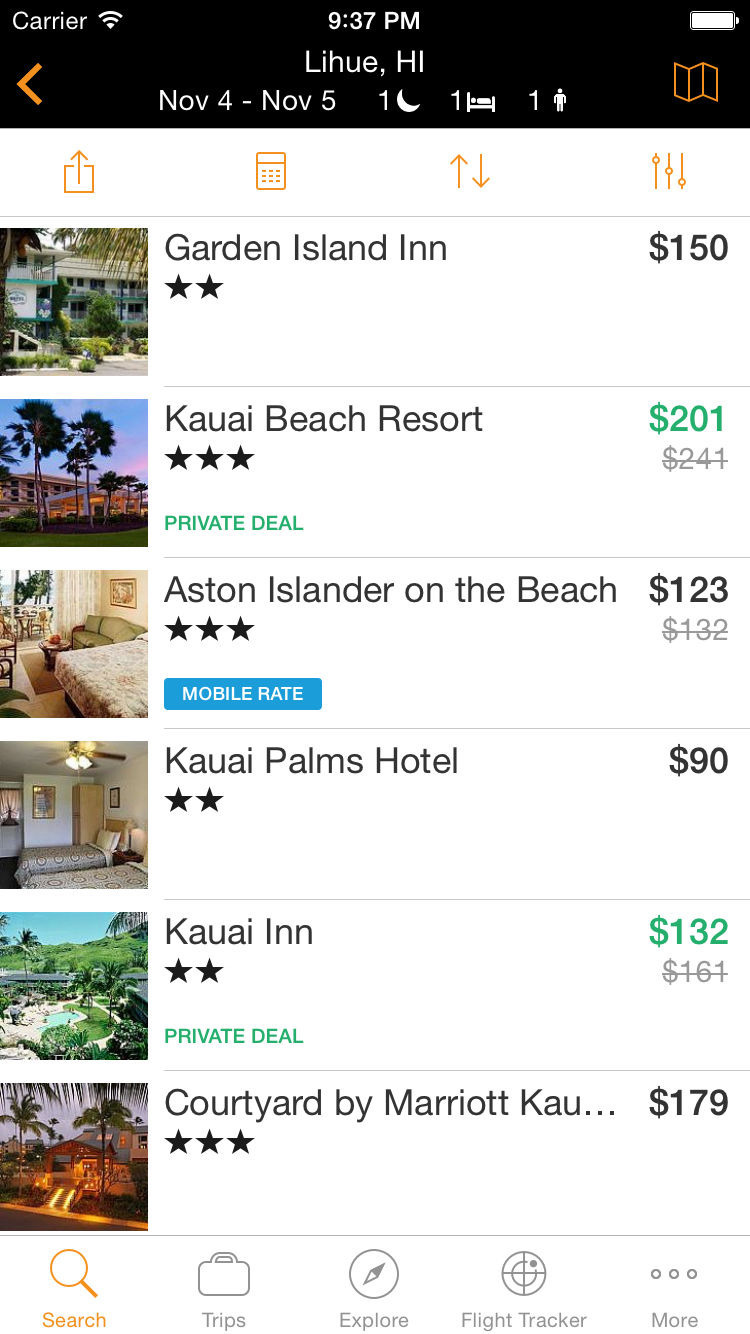Screenshot of a phone displaying hotel search results for accommodations in Kauai, Hawaii. The phone shows full carrier signal at 9:37 PM, with a full battery indicator. The search results are for a one-night stay from November 4th to November 5th for one person requiring one bed.

1. **Garden Island Inn**:
   - Price: $150 per night
   - Rating: 2 stars
   - Image: Tropical garden background

2. **Kauai Beach Resort**:
   - Price: $201 (on sale from $241)
   - Deal: Private deal
   - Image: Front view of the hotel

3. **Aston Islander on the Beach**:
   - Price: $132 (mobile rate)
   - Rating: 3 stars
   - Image: Room with a green couch and flower-printed décor

4. **Kauai Palms Hotel**:
   - Price: $90
   - Rating: 2 stars
   - Image: Basic room with two small beds

5. **Kauai Inn**:
   - Price: $132 (down from $161)
   - Deal: Private deal
   - Image: Foliage with an open pool

6. **Courtyard by Marriott Kauai**:
   - Price: $179
   - Rating: 3 stars

The bottom of the screen features a yellow search bar, with icons for trips (briefcase), explore (compass insignia), and a flight tracker (targeting system with radar dot). Three dots indicate more options. The user appears to be searching for suitable lodging options in Kauai, Hawaii.